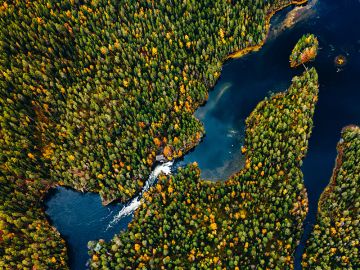This aerial photograph, captured from approximately a thousand feet in the air, showcases a densely forested lake system with interconnecting landmasses. The landscape is predominantly covered with medium to dark green trees, interspersed with a small percentage of yellow and orange foliage, suggesting an early spring setting. The scene features a jagged coastline and multiple water inlets that narrow and widen in various places. 

At one end, the waterway starts as a narrow segment that broadens into a large bay area featuring an island at its mouth. A narrow section with visible white-capped water potentially indicates a waterfall, where water transitions from a higher area to a lower one before expanding into a large oval-shaped body of water. This larger water body extends off the lower portion of the image. On the right side, a peninsula juts into the water, creating another cove where the water encircles back into the landmasses. This intricate system of waterways and forested peninsulas paints a complex and beautiful portrait of nature from above.